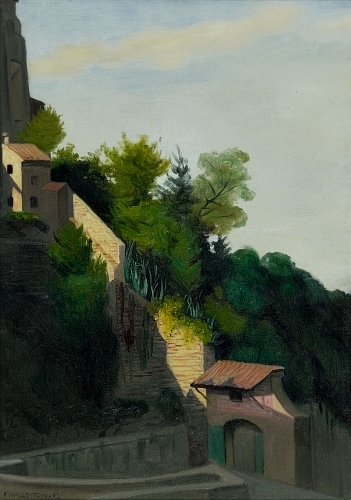This detailed oil painting captures a scenic outdoor setting during the late afternoon, rendering a serene and timeless ambiance. Dominating the foreground is a historic structure with an arched doorway, possibly reminiscent of an 1800s garage or an ancient edifice, adorned with a rust-colored gabled roof and flanked by greenery. To the right, a stone fence encircles the building, further enhancing its old-world charm, and leading the eye upwards through the composition.

Rising towards the upper left section of the canvas is a sloping hill dressed in lush green grass and thriving with dark and light green trees contrasting against a rich blue sky dotted with white clouds. Atop this hill rests a significant dark gray structure, possibly a church or cathedral, recognized by its steeple-like appearance and a striking gabled roof, adding a touch of architectural grandeur to the scene. The landscape evokes the timeless streets of Rome with its blend of architectural beauty and verdant foliage. The intricate details and the harmonious interplay of colors in this oil painting create a vivid portrayal of pastoral serenity and historic elegance, quite devoid of any textual interruptions.